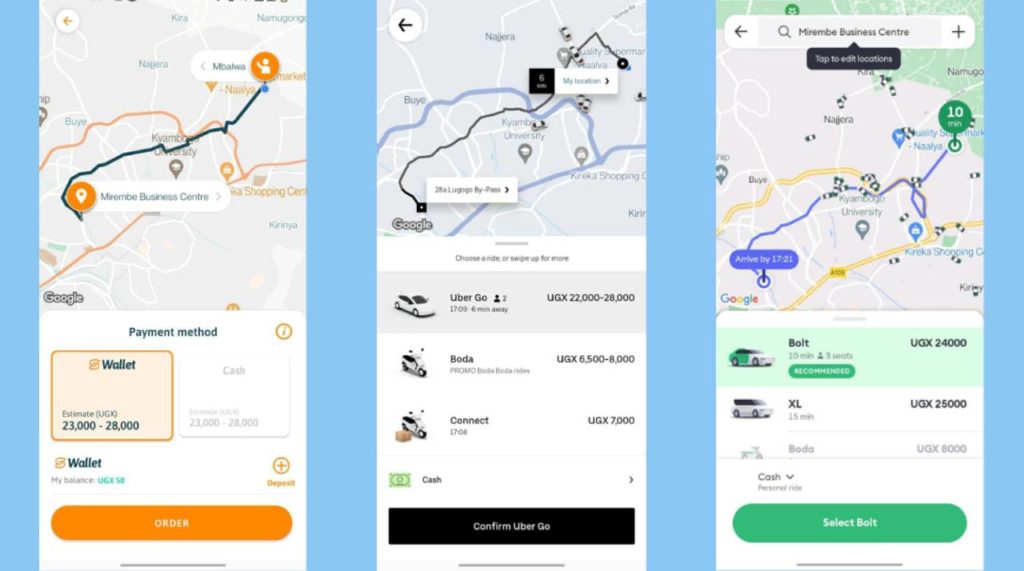In this triptych of images, each appears to be associated with a ridesharing service, possibly Uber or a similar platform.

1. **First Image**: This graphic features a predominantly white and black interface accented with orange. It resembles a payment screen, displaying details such as "Payment Method: Wallet" and a monetary range from UGX 23,000 to UGX 28,000. The graphic also includes an orange button labeled "Order."

2. **Second Image**: The central graphic clearly pertains to Uber. It presents a grayscale map with a black route line and small white cartoon car icons. The interface showcases various Uber ride options like Uber Go, Boda, and Connect, each with corresponding prices listed in black text. At the bottom, a black button labeled "Confirm Uber Go" in white text is prominently displayed.

3. **Third Image**: This image also displays a map, featuring gray and green tones. Similar to the previous image, it includes white cartoon car icons and a Google logo, indicating that all three maps utilize Google Maps. This screen lists rideshare options such as Bolt for UGX 2,460 and XL for UGX 25,000. A green button with white text that reads "Select Bolt" is present.

Each graphic conveys a different aspect of the ridesharing experience, from payment options to choosing your ride on a map interface.